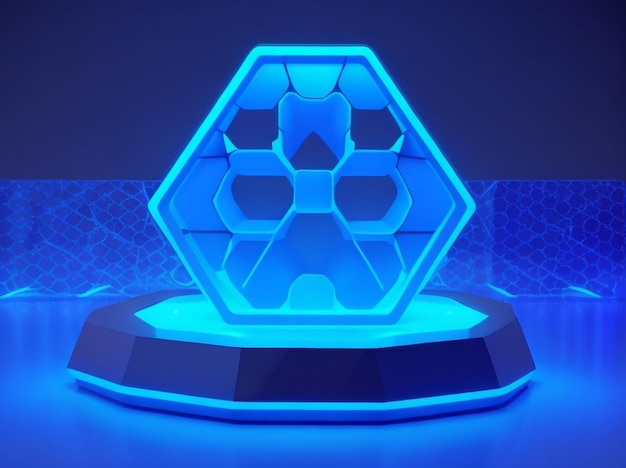The image showcases an intricate, futuristic glass-like structure beautifully lit by a blue neon light emanating from a monochromatic black base. This six-sided geometric marvel, somewhat resembling an award or a sophisticated modern decor piece, features several see-through cavities that accentuate its unique shape. The base is also composed of glass elements and is central in illuminating the entire setup. Surrounding the main structure are additional geometric shapes that form a visually captivating wall, further highlighting the detailed and elaborate design. The dominant color throughout the composition is blue, with various shades from light neon to dark, creating a mesmerizing contrast against the dark surroundings. This scene projects a distinctly modern and holographic feel, with the lit-up structure being the focal point in this strikingly dynamic and detailed display.